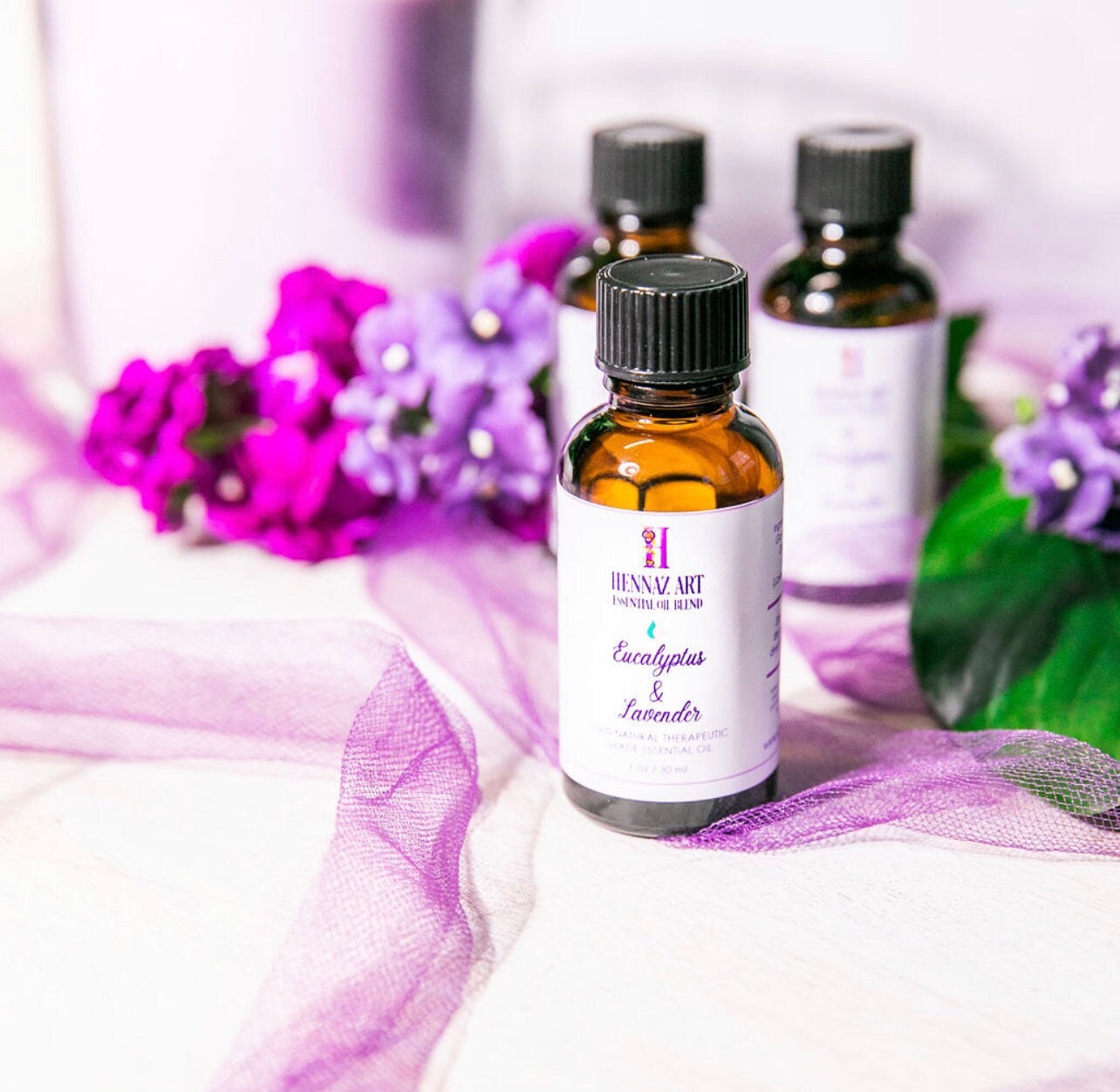This indoor photograph captures a beautifully arranged scene featuring three small brown essential oil bottles with black twist caps and white labels, centered against a white backdrop and tablecloth. The bottles, reminiscent of old medicine containers, are embossed with the name "Hennaz Art" in purple cursive atop the label, with the visible bottle distinctly labeled as an "eucalyptus and lavender oil blend." The foreground bottle is in sharp focus, while the two in the background are slightly blurred. The tabletop is elegantly decorated with strands of purple tulle, purple lace, and a scattering of purple flowers with yellow centers and dark pink flowers. Some of the flowers are interspersed with green waxy leaves, mostly visible on the right-hand side of the image. In this richly detailed composition, the primary colors of purple, brown, black, green, and white merge harmoniously to create an inviting and fragrant visual display.